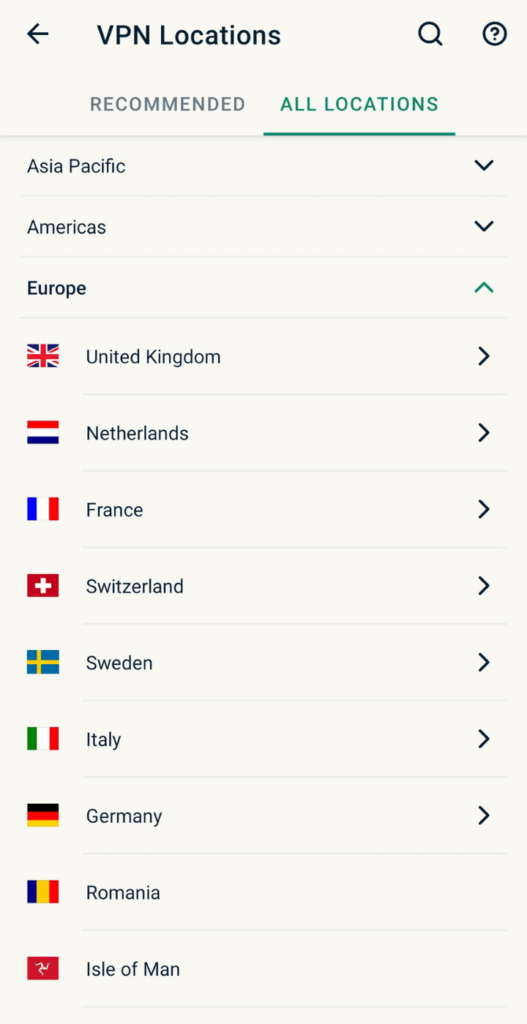The image showcases a web page with a predominantly grayish color scheme, focused on displaying various VPN locations. At the top, the header "VPN locations" is prominently featured, with a left-pointing arrow icon beside it. Adjacent to the header are a search icon and a question mark icon.

Below this header, there are two tabs: "Recommended" in gray and "All Locations" in green, with a green bar underscoring the currently selected "All Locations" tab. 

The main content is a structured list categorized by regions, with each section indicated by an arrow. The "Asia-Pacific" and "Americas" sections are marked with downward-pointing arrows, while the "Europe" section stands out uniquely with a bold font and an upward-pointing arrow in green.

Within these regions, individual countries are listed alongside their respective national flags, displayed on the left side of the country names. 

For the "Europe" region:
- United Kingdom: Right-pointing arrow
- Netherlands: Right-pointing arrow
- France: Right-pointing arrow
- Switzerland: Right-pointing arrow
- Sweden: Right-pointing arrow
- Italy: Right-pointing arrow
- Germany: Right-pointing arrow
- Romania and Isle of Man: Display their flags but notably lack any directional arrows, a unique feature in this list.

The overall design is straightforward and functional, albeit somewhat bland in appearance, with Europe notably distinct due to its bolded font and different arrow direction.